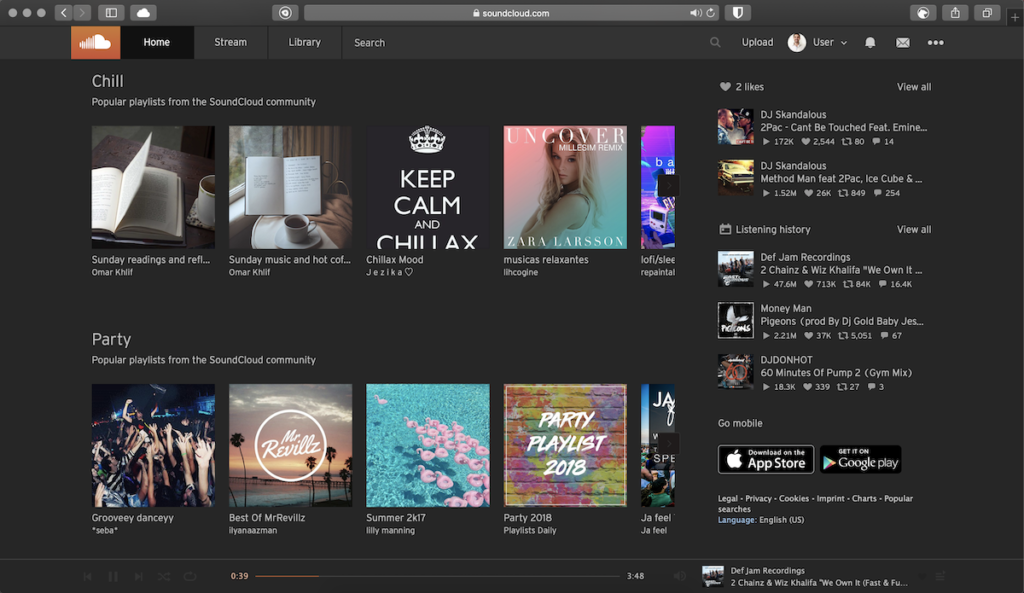The image is a screenshot of a SoundCloud webpage, predominantly rendered in shades of black and gray with splashes of color from various album covers. At the very top, there's a search bar, accompanied by a lock icon, indicating that the URL, soundcloud.com, is secure. Adjacent to the search bar are icons for a speaker with volume control and a refresh button.

On the top-right corner, a shield icon further signifies the site's security. Additionally, there's a cloud icon with an orange background that represents the SoundCloud logo. The main navigation menu is displayed on the left side, featuring options labeled Home, Stream, Library, and Search.

In the user's activity section on the right, there is a heart icon showing two likes. Below it is a playlist featuring "DJ Scandalous," followed by "Tupac - Can't Be Touched featuring Eminem," and "DJ Scandalous, Method Man featuring Tupac and Ice Cube." 

The Listening History section includes entries such as "Def Jam's Recordings," "Money Man," and "DJ Don Hot." 

There are multiple playlists listed with vivid album covers, including:
- Chill Playlist: A popular collection from the SoundCloud community.
- Sunday Readings: A playlist designed for mellow, Sunday listening.
- Keep Calm and Chillax: Featuring "Uncover," a cover by Zara Larsson.
- Party Playlist for Groovy Dancy: Energizing tracks for a dance mood.
- Best of Mr. Revels.
- Summer 2017.
- Party 2018.

The colorful album covers lend vibrancy to the otherwise monochromatic page, showcasing a diverse array of music and playlists designed to cater to different moods and activities.